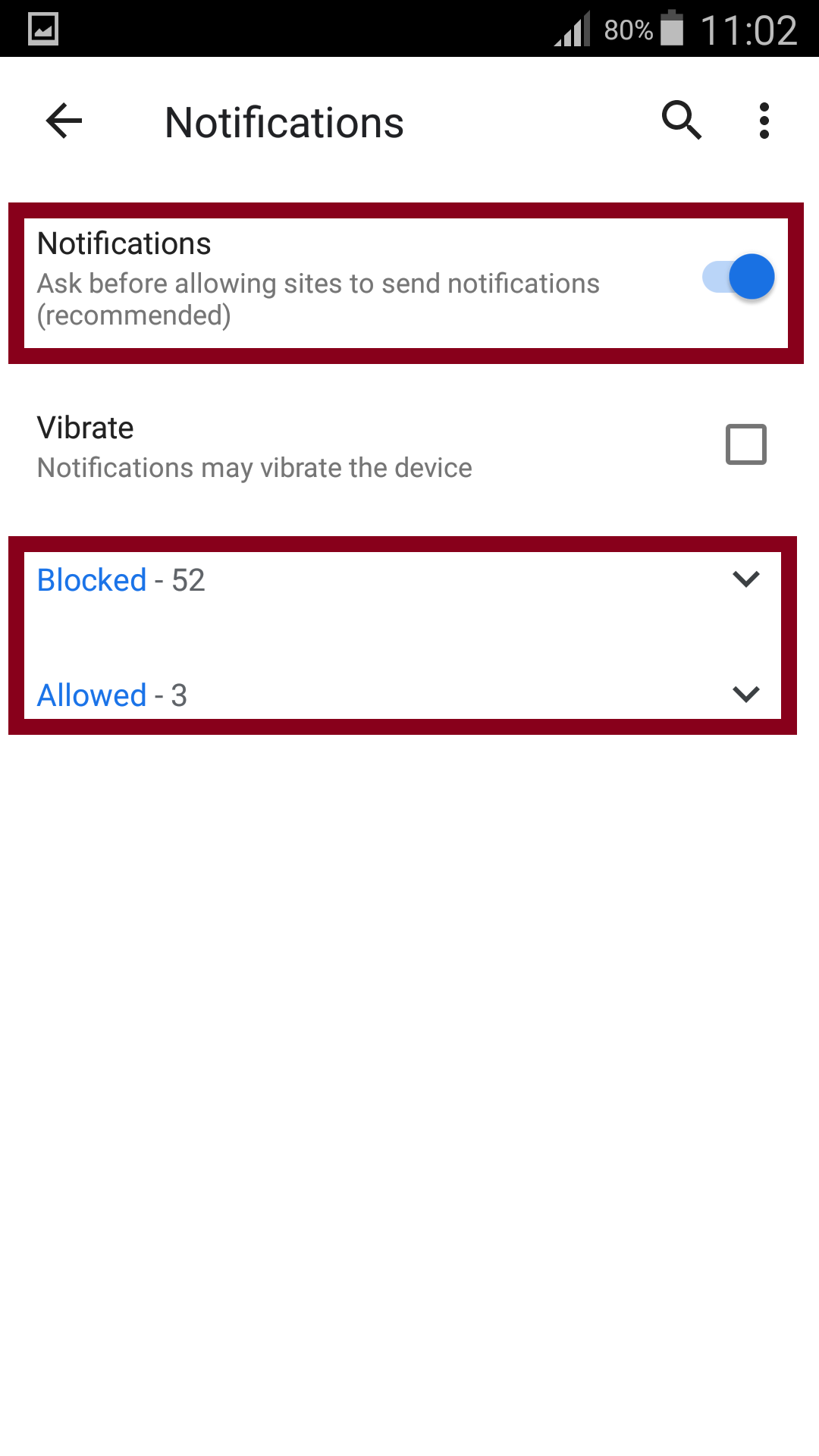In this detailed image of a cell phone's screen, a website interface is prominently displayed. At the top right corner of the screen, nestled within a black bar, the time is shown as 11:02. The battery indicator reveals approximately 80% charge with three out of four bars illuminated. Adjacent to the battery icon is a small box image indicating signal status.

Below this black bar, the interface features a notification settings page. On the top left, there's a label that says "Notifications" followed by an arrow pointing to the left. The top right corner displays a search icon alongside three vertically aligned dots, suggesting additional settings or options.

Dominating the middle of the screen, a maroon-colored box outlines a rectangle with the heading "Notifications." In gray text, it states, "Ask before allowing sites to send notifications," with a recommendation note. Next to this text is a blue circular toggle, indicating an option that can be activated or deactivated by sliding.

Beneath this notification setting, a white section provides additional options. It reads "Vibrate," with an explanation that notifications might vibrate the device. An unchecked box is present next to this text, allowing the user to enable or disable this feature.

Below the white section, another maroon-colored box contains more settings. The box displays "Blocked 52" in bold text. Below, two sections, "Blocked" and "Allowed," are highlighted in blue, each accompanied by a count and a drop-down arrow to view or modify the respective lists. The "Blocked" section shows 52 items, whereas the "Allowed" section displays 3 items, each with the functionality to expand for further details.